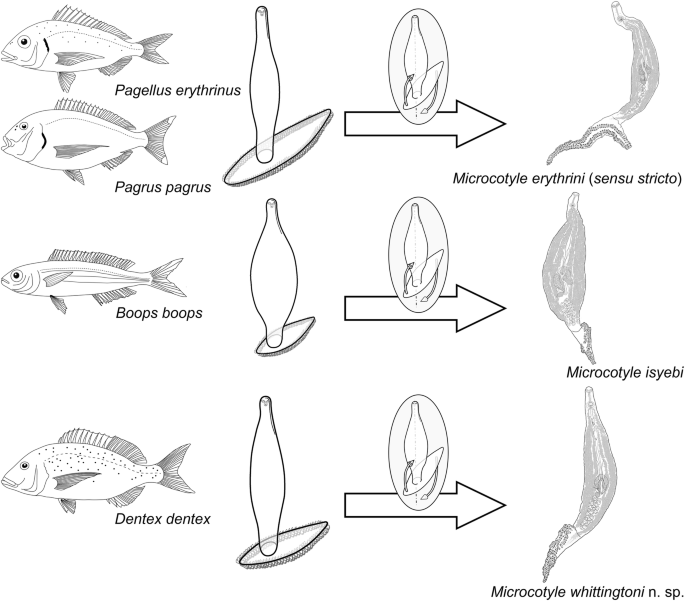This black and white scientific illustration resembles a flowchart and displays a detailed examination of different species of fish and their corresponding biological entities. The diagram is organized into three distinct rows, each row associating a fish on the left with an organism on the right through an intermediary object resembling a vase or bottle. 

In the first row, the fish at the top is labeled "Pagellus erythrinus." An arrow from a vase-like structure points to an organism identified as "Microcaudal erythrina (Sensu stricto)." The second row presents a fish named "Boops boops," with a similar vase object and an arrow leading to "Microcaudal Isiabeb." In the third row, the fish "Dentex dentex" is connected via an arrow from the vase-like object to an organism labeled "Microcaudal Wittingtoni."

Each fish in the left column is presented with its scientific name: "Pagellus erythrinus," "Boops boops," and "Dentex dentex." In summary, the illustration appears to be a scientific analysis, systematically charting the relationship between these fish species and various micro-organisms through visual links signified by the vase-like symbols and directional arrows.